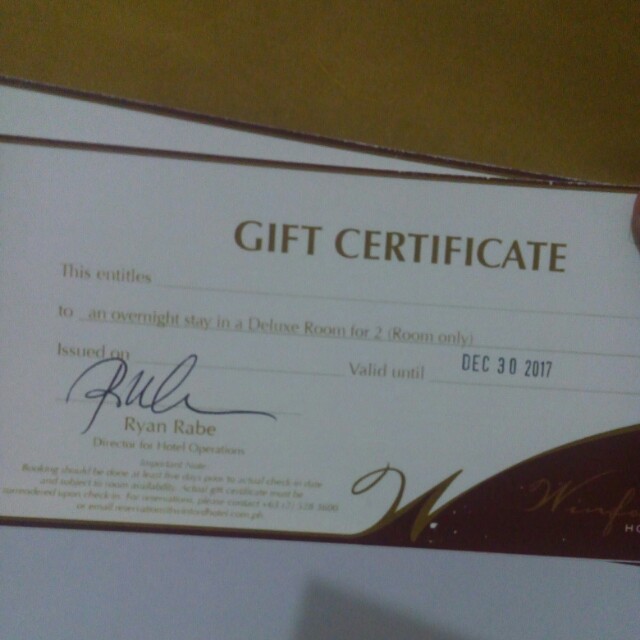The photograph prominently features a white gift certificate for an overnight stay in a deluxe room for two, issued by a hotel. The certificate's text is rendered in gold, with "Gift Certificate" prominently displayed at the top. Below this, it includes fields for customization, some of which are filled in: the recipient, the type of stay, the issuing date, and an expiration date. Specifically, the offer is valid until December 30, 2017, stamped in a different font. A blue handwritten signature of Ryan Rabe, the Director of Hotel Operations, is present above his printed name. The photograph also reveals another partially obscured gift certificate beneath the featured one, all against a brownish background, which may be a table or flooring. The hotel's logo is partially visible in the bottom right corner but is cut off, leaving it indistinct.